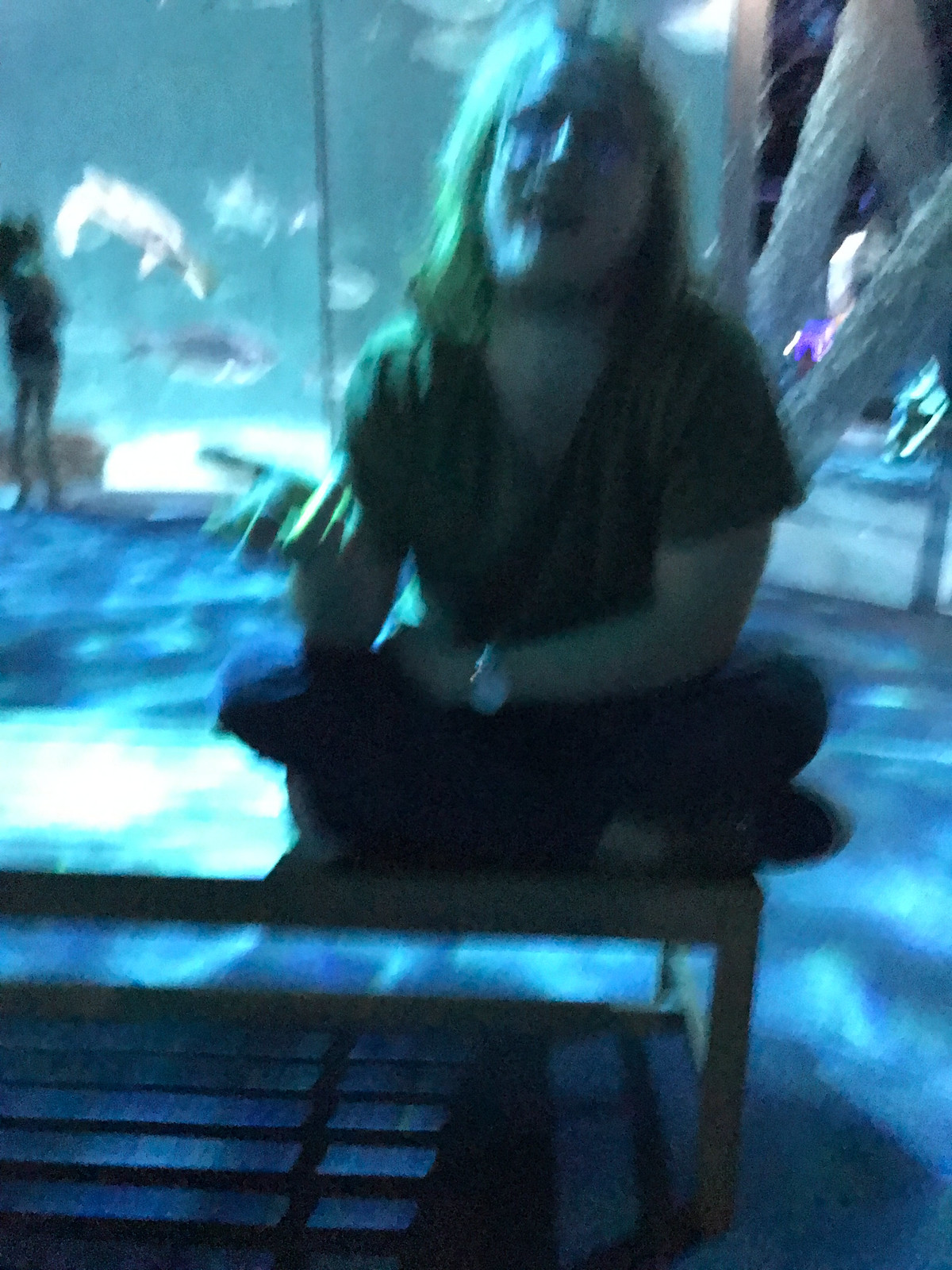In this photograph, which is very blurry and out of focus, a man with shoulder-length blonde hair and fair skin is seated cross-legged on a plain bench inside an aquarium. He faces the camera, wearing a dark v-neck t-shirt and long pants with dark canvas sneakers featuring a white rubber border. The man wears a wristwatch with a large circular face on his left hand. His right arm is outstretched towards the camera, and his facial features are indistinguishable due to the blur, though his mouth appears slightly open, suggesting he might be mid-speech or laughing. Behind him, large floor-to-ceiling windows reveal an aquarium tank teeming with marine life, including large fish and possibly a dolphin. To the left, a small child stands transfixed by the aquatic display, while the bluish floor of the aquarium, patterned with splotches of light, reflects the underwater atmosphere.